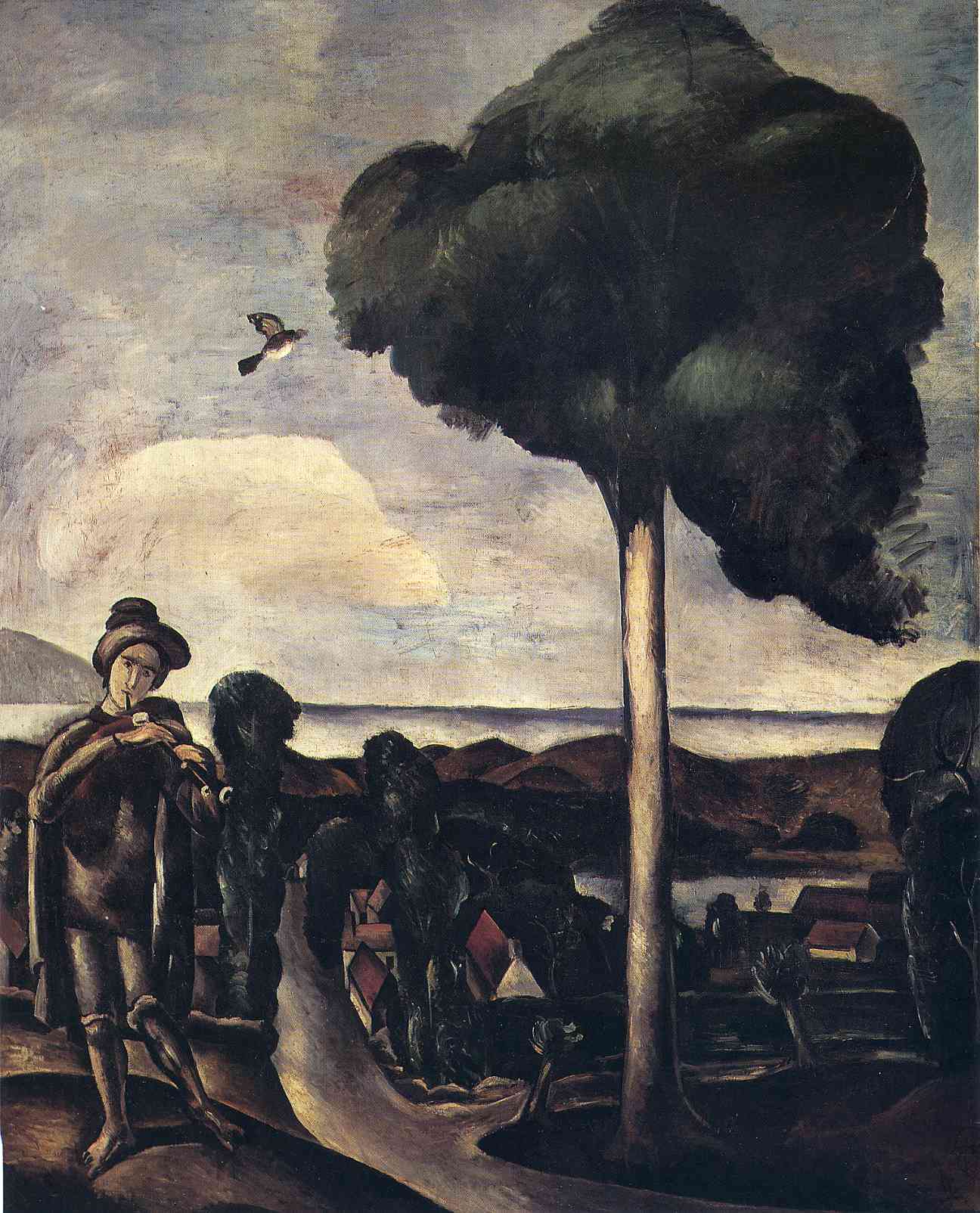The painting, "The Bagpiper at Khmers" by Andre Duran, is a vertical rectangular composition that exudes a dark, enigmatic atmosphere. Dominating the right side, there is a tall, smooth tree with foliage resembling a dense, dark cloud. To the left of this tree, a small grayish bird with a white underbelly is captured mid-flight, possibly heading towards the tree to nest or rest. Below, the landscape transitions into a shoreline where faint figures of people are discernible; among them, a standout figure is a bagpiper, or possibly an oboist, standing barefoot on a hill. This character is described with detailed attire, including a hat, cape, and what appears to be armor, and is absorbed in playing a dark, elongated instrument. The person has their hair styled in a bun. The background reveals a vast expanse of water with a dark surface, leading up to a sky that exhibits a gradient from dark blue with hints of purple and red near the horizon, punctuated by a single prominent white cloud on the left. The overall scene is enveloped in a mixture of dark greens, browns, and the occasional splash of red, creating a compelling contrast between the detailed foreground and the somewhat vague, dreamy background elements including water and distant buildings.